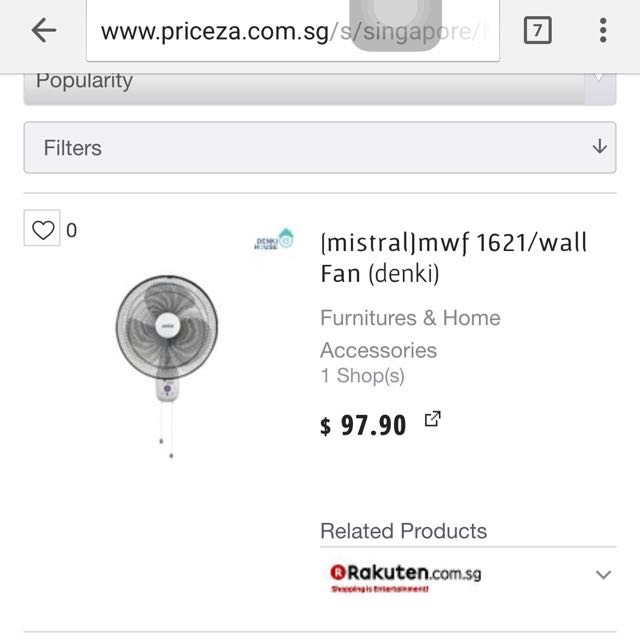Detailed Caption: 

The image showcases a simple wall-mounted fan encased in a protective cage with three propeller blades. Two pull chains dangle from the fan, likely used for adjusting settings. To the right of the fan, the brand name "Mistral" and model number "MWF 16/1" are prominently displayed. This suggests it's a model designed for wall installation, possibly including brackets for mounting. 

The control options seem to include settings for oscillation and fan speed toggled between high and low. The product falls under the "Furniture" category and is listed with the accessory sub-category. The price for this fan is marked at $97.90, and there's a button to purchase it through a third-party site. 

Below the price, there is a section for related products indicating Racket Tunes as an alternative vendor, likely offering similar fans at competitive prices. The webpage hosting the image of the fan seems to be zaa.com, displaying its interface with a search bar at the top, a left arrow for navigation, a filter dropdown, and a sort-by-popularity option. Additionally, multiple tabs are open in the browser, visible next to the search bar, and there are also settings depicted by three dots and a subscription box.